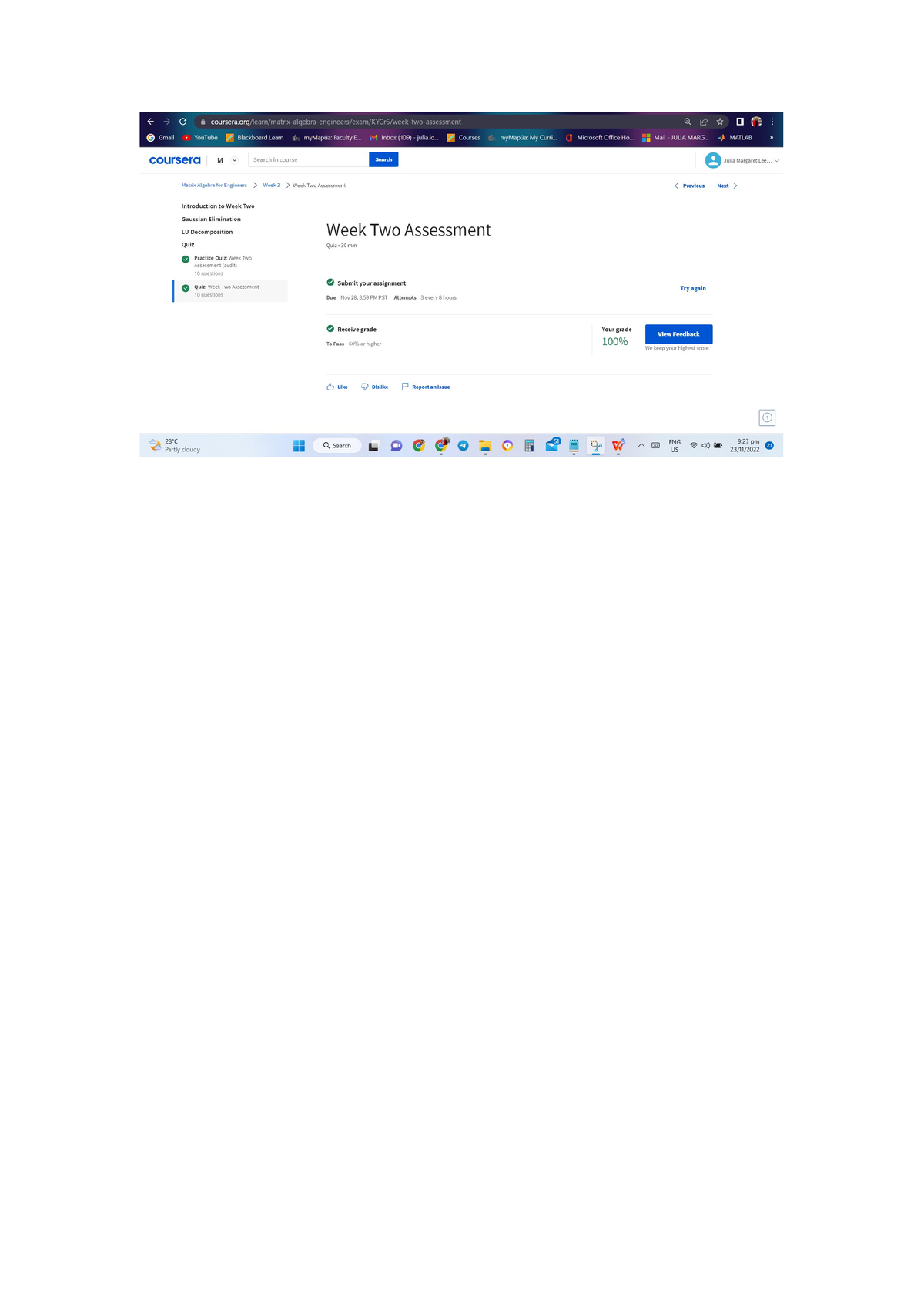The image is a small website screenshot with a sophisticated color scheme dominated by shades of blue. The header features a dark black box running across the top. The background showcases a gradient transition starting with teal, flowing into black, purple, black again, teal, black, and ending in purple, finally returning to black as the pattern repeats.

On the right and left sides of the screen, a variety of icons are visible. Among the colors, there are striking hues of red and yellow. Beneath the gradient background, the word "Courses" can be discerned in blue text, albeit faintly.

Prominently at the top, there is a blue box housing a generic profile picture of a person. Adjacent to the profile picture, the text "Two-Week Assessment" is displayed, accompanied by green circles and black writing alongside it. Below this section lies more text, situated above a blue solid box with white text inside.

At the bottom of the image, a gray bar stretches horizontally with a multitude of icons adorning it. These icons are of various colors, including Google's recognizable color palette, pink, and many shades of blue. The icons come in different shapes and sizes, each indicating a distinct function or feature. On the left side of the screen, additional text descends from underneath the word "Courses," providing further details.

This detailed depiction conveys the intricate layout and color coordination of the website's design elements, capturing its distinctive aesthetic.